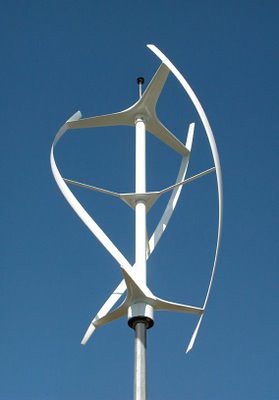The image showcases a tall, white, metal structure set against a clear blue sky, casting some shadows. It resembles a unique, modern wind turbine with an artistic twist. The central element is a long white pole anchored with a black pin at the top. Near the top of this pole, there's a triangular plate from which three horizontal lines extend outward at the same level. At the end of each horizontal line, a vertical arc-shaped blade curves upward, creating a spiral or boomerang-like design. These white, metallic arcs contribute to a swirling visual effect, giving the structure an aesthetic appearance even when stationary. The entire setup exudes an architectural elegance, blending functionality with a sense of dynamic motion.